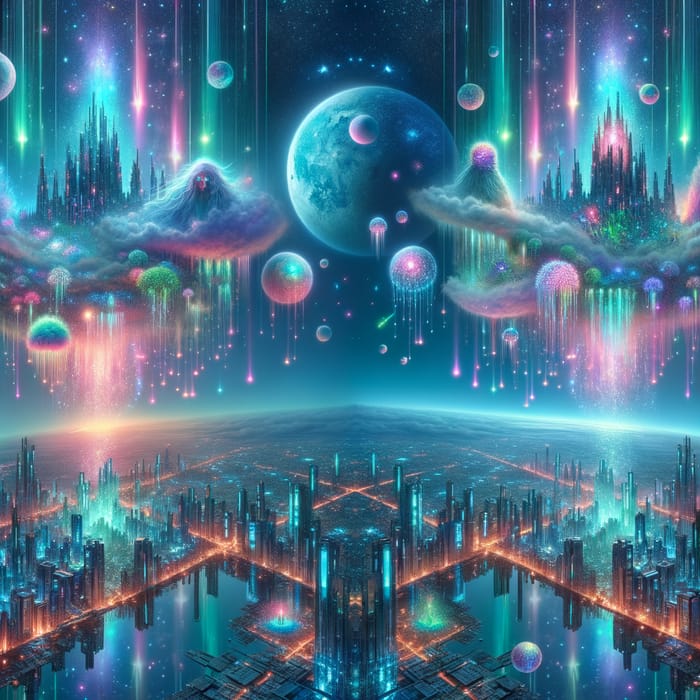The image features a mesmerizing futuristic digital illustration dominated by light blue, pink, and purplish hues with intricate details. At the top half of the image, a large globe resembling a moon looms in the background, casting a celestial glow. Surrounding this central globe are smaller circle globes, accentuated with white lines highlighted in pastel blue and pink. Clouds, with spiky formations extending upwards, frame the left and right sides of the scene. Below, an eye-catching horizon marked by a pointy center separates this upper part from a sprawling futuristic cityscape below. This city, seen from a floating aerial view, is rich with tall buildings that glow blue, green, and pink, conveying a pastel ambiance. Mirrored structures create an enigmatic effect, while an orange-gold grid of crossing lines adds a sparkling intricacy just above the horizon. The image seamlessly blends elements of a terrestrial city with grand, castle-like edifices, all illuminated by vibrant lights, creating an otherworldly, yet harmonious, visual masterpiece.